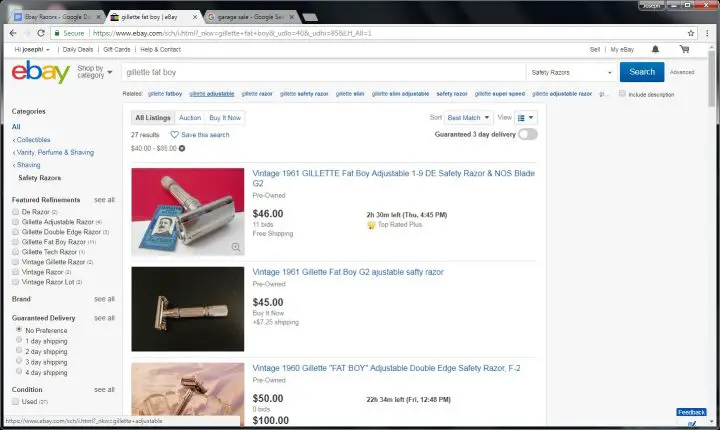Screenshot Description: 

A user conducts a search for "Gillette Fatboy" on eBay, resulting in 27 listings primarily showcasing vintage Gillette Fatboy razors. The search results feature prominently three top-rated pre-owned razors priced at $46, $45, and $50, respectively. Each listing offers an option for guaranteed 3-day delivery. The user did not apply specific preferences for guaranteed delivery or any additional filters. However, the search results are sorted by "Best Match", which is indicated as the sole filtering criterion used. Various filter options are available for narrowing down the search, including categories like Gillette Adjustable Razor, Vintage Razor, and Brand. Users can also filter results by delivery guarantees, condition, and purchasing options such as "All Listings" or "Buy It Now". The search interface allows saving search results for future reference.